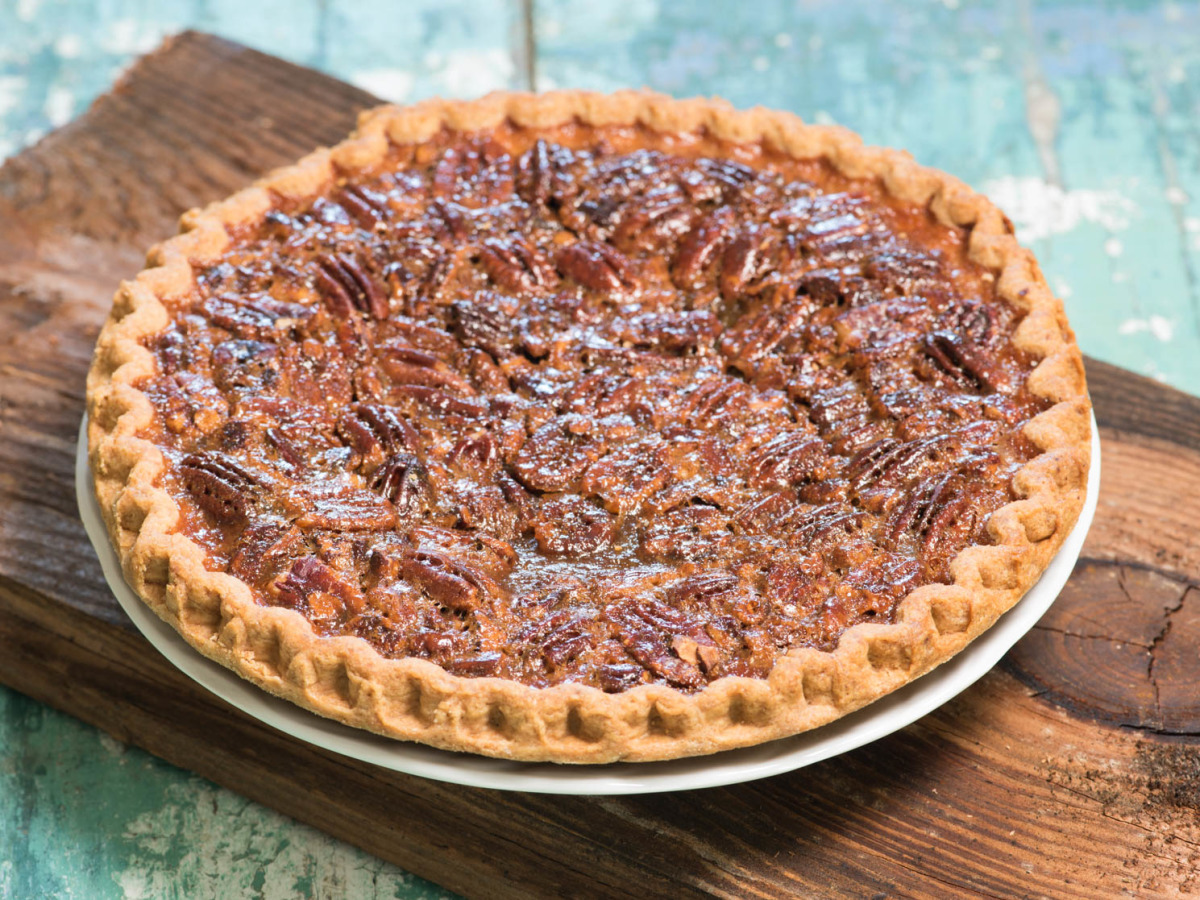This detailed color photograph, taken from above, showcases a full pecan pie sitting in a silver pie dish with a pinched, wavy light brown crust. The top of the pie is a glossy, dark brown, densely packed with shiny, candied pecans that cling together. The pie rests on a wooden board, which is positioned on a green surface adorned with patches of white and light blue scuffs, resembling a weathered picnic or park bench. The image captures the pie’s rich textures and colors, with the contrasting settings providing a rustic backdrop. The photograph is in a horizontal and rectangular format.